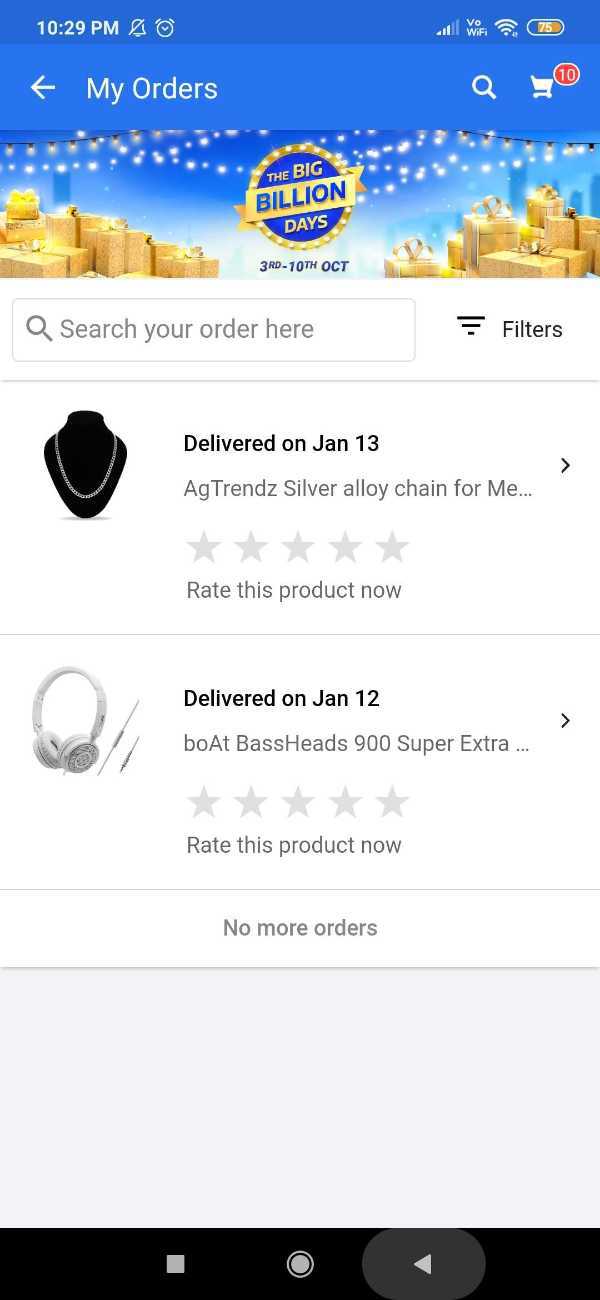This screenshot, taken from a person's cell phone, displays an interface loaded with details. At the top, there is a dark blue border containing essential information: the time (10:29 PM) and the battery status (75% charged). Below it, a lighter blue border features a back arrow, the text "My Orders," a magnifying glass icon for search, and a shopping cart icon adorned with a red circle indicating 10 items.

The main section of the screen showcases an image of white fairy lights elegantly strung up, casting a gentle glow on piles of gold-wrapped packages tied with gold bows. A circular seal with white lights around the edge stands out in the center, announcing "The Big Billion Days" event from the 3rd to the 10th of October. Directly below the image, there is a search bar prompting users to "search to order here."

The content further includes two product descriptions. The first is a photograph of a silver chain displayed on a black stand, marked as delivered on January 13. It is described as a "Black Trends Silver Alloy Chain for Men," with a prompt to rate the product and five empty stars awaiting user feedback. The second product is an image of white headphones, delivered on January 12, identified as "BOAT Bassheads 900 Super Extra," also accompanied by five blank stars and a call to rate the item. The screen concludes with a simple statement: "No More Orders."